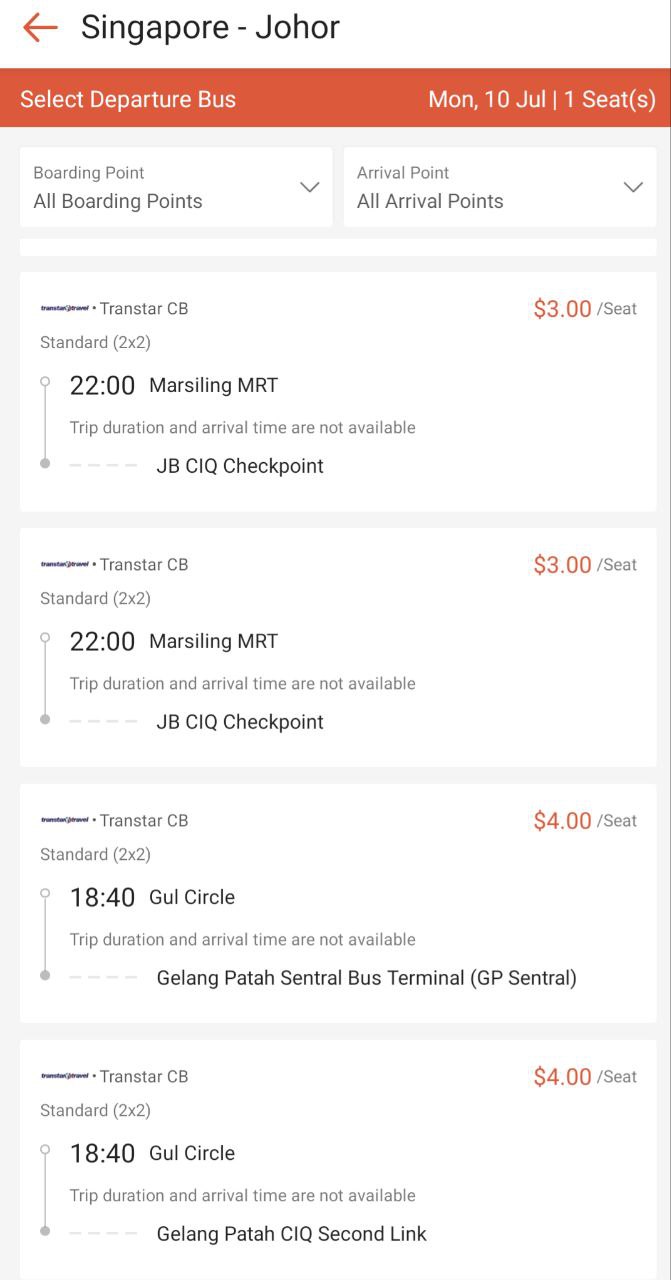A mobile screenshot captures the detailed departure times and information for a bus trip. Displayed prominently at the top, the date is Monday, 10th of July, and the trip is booking one seat. Just beneath this date bar, there's a filter section where users can choose from various boarding and arrival points or select 'All Boarding Points' or 'All Arrival Points.' 

The screenshot lists four available bus trips, each detailing the departure date and time, the type of trip, the checkpoint or destination, and the price per seat. Prices for these trips are either $3 or $4 per seat. The user interface is clean and basic, featuring a very traditional layout. The service is specifically for the route between Singapore and Johor.